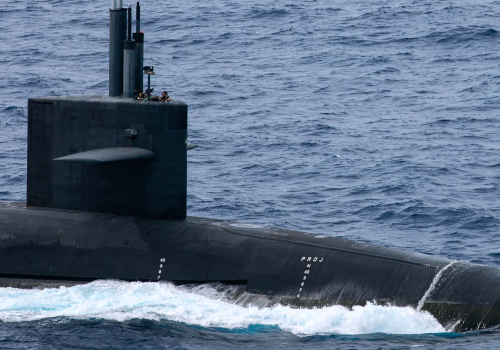The photograph captures an ocean scene with choppy, deep blue water and small, scattered waves. Dominating the foreground is a large, black submarine, partially submerged and spanning across the entire width of the rectangular image. The submarine features a small tower on top, along with several pipes protruding from it. Around the base of the submarine, the water is particularly turbulent, forming white caps and frothy white suds where the waves crash against its hull. The side of the submarine displays barely discernible letters, "P-A-D-J," and small windows. The overall scene conveys a sense of motion as the submarine appears to be heading east through the rough sea.